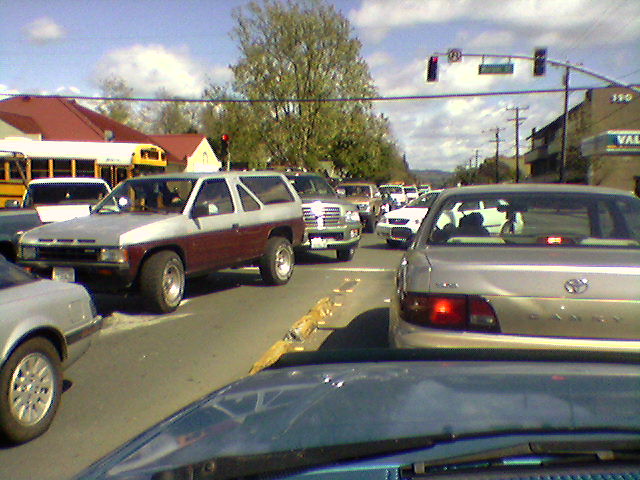The photograph captures a congested intersection from the perspective of a car's driver's seat, looking over the blue hood and windshield. In the center foreground, a silver Toyota Camry is prominently visible. A silver curved pole with a red traffic light stands on the right side of the frame. The sky is clear blue adorned with sporadic white clouds. In the background, a brown building is visible on the right, while a white building with a red roof stands to the left. The intersection itself is cluttered with various vehicles, including a school bus, a silver and red two-tone SUV, a silver pickup truck, and a white car, all merging and blocking the roadway. The scene epitomizes a typical traffic jam in an urban setting.